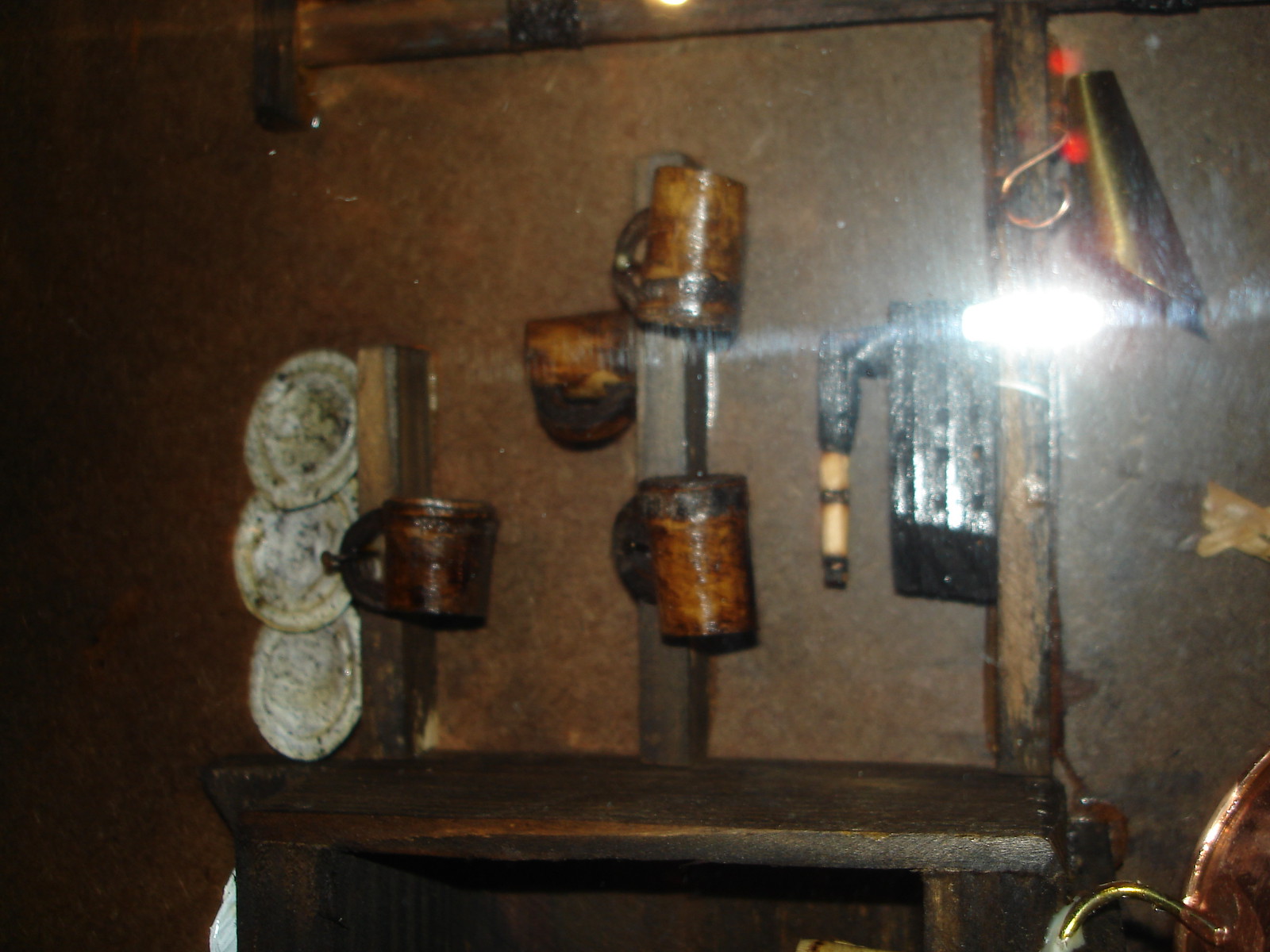This photograph, taken from the inside and slightly blurry with a flash reflecting back, captures a detailed arrangement against a brown wall. Centered in the scene is a wooden bench extending across the length of the image. Above the bench, various items are meticulously organized on wooden boards and slats. 

On the left end of the bench, a board mounts three white plates, possibly dirty, hanging closely together. Beside them, a tin cup or mug dangles sturdily. Moving right to the center, another vertical board showcases three ceramic mugs: one inverted at the top and two positioned on either side. The far right end features a taller board, though a bright light obscures the specifics of the implements hanging there, rendering them indiscernible. Interspersed among these implements are hints of copper objects with spouts, adding metallic accents to the scene. The entire setup, nailed securely to wooden slats, emphasizes a rustic yet organized display of ceramic and metal paraphernalia.